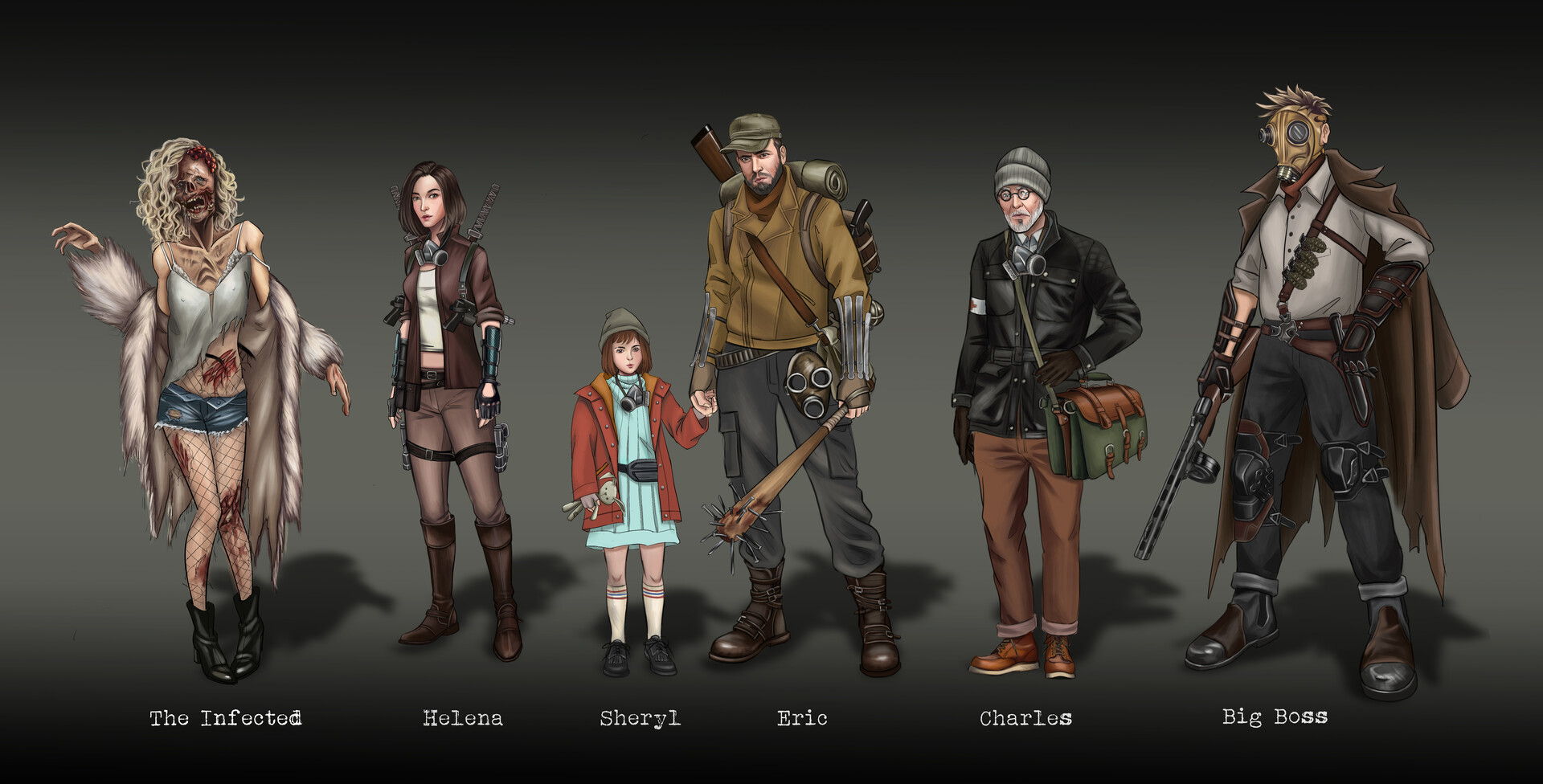The image showcases a row of six distinct video game characters aligned across a background that transitions from a medium gray to a darker shade along the top and bottom edges, with shadows emphasizing the figures. On the far left is a thin woman, labeled "The Infected" in white text beneath her. She wears short shorts, a fur coat, and boots; her face is largely decayed, typical of a zombie. Next to her stands a woman in a black leather jacket, leather pants, and boots, equipped with numerous weapons. This character is identified as Helena.

In the center of the lineup are a little girl named Cheryl and a man named Eric. Cheryl is depicted in a blue dress and a red overcoat with a stocking cap, while Eric, who holds her hand, wears a bomber jacket, cargo pants, military-style boots, and a knit cap. Eric is heavily armed, with a spiked club at hand, a backpack, and bedrolls, indicative of a rugged survivor. 

To their right is Charles, described as an elderly man dressed in a black leather jacket, brown pants, and a knit cap, also carrying a large bag that suggests he's prepared for an apocalypse. 

On the far right stands the figure labeled "Big Boss," wearing a distinctive gas mask and a Dracula-like brown cape over a light gray shirt. This character, also armed to the teeth, is defined by his ominous appearance and readiness for battle, underscored by a weapon-laden outfit featuring a white button-down shirt and a glove. All characters are depicted with a sense of readiness and survival within a dark, foreboding atmosphere.